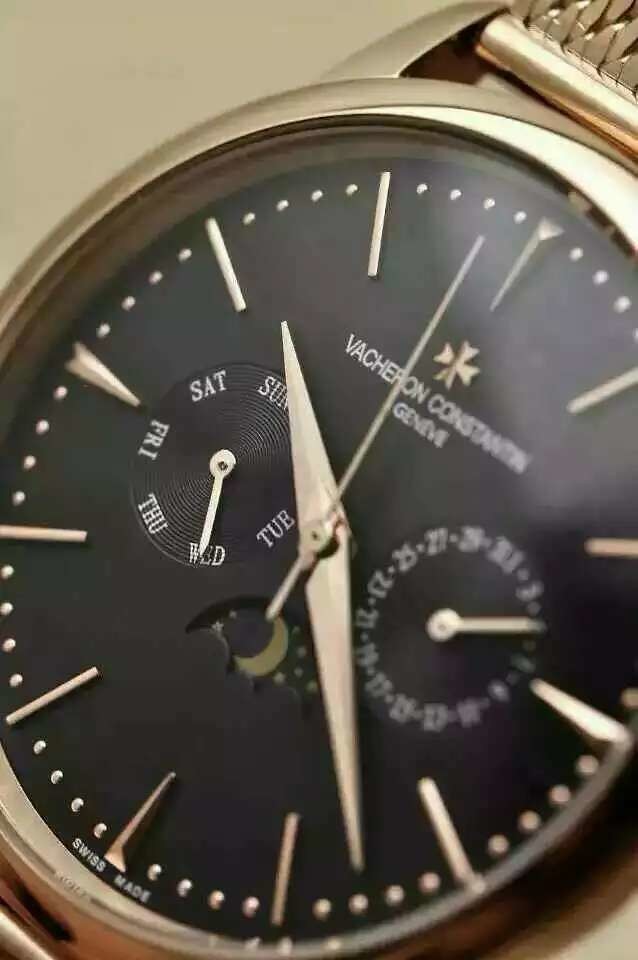A luxurious gold watch rests elegantly in the center of a light beige table. The watch features a polished gold head paired with a sophisticated, gold braided band that adds an element of intricate craftsmanship. The black face of the watch is striking, adorned with minimalist gold markers in the form of straight lines, rather than traditional numbers. Complementing the markers, the hands are also gold, ensuring a harmonious design. The watch face includes white lettering, providing clear, crisp details of the day and date, enhancing both its functionality and style.